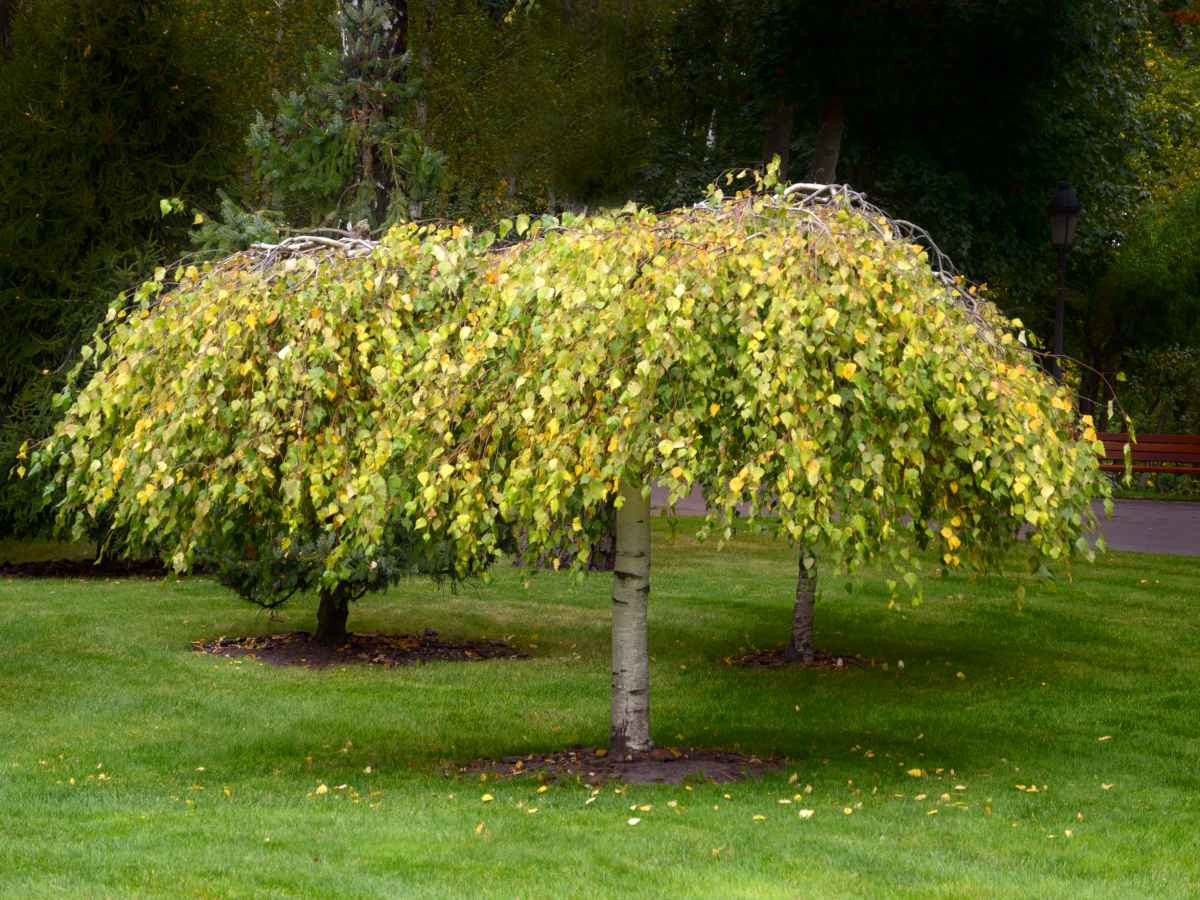The image features a serene park scene centered around a unique, low-profile, weeping-style tree with a striking white bark trunk. This narrow, cylindrical trunk rises with little tapering, leading to a canopy where densely packed branches sweep outward and downward, creating a wide, horizontal expansion with light green to yellowish leaves. The tree's leaves, indicative of changing seasons, are heavily clustered on the branches, which extend to about halfway down the trunk, resembling a weeping willow. Surrounding the tree, the well-manicured, dark green grassy lawn adds to the serene atmosphere. A wooden bench and a streetlamp can be seen in the background, further highlighting the park setting. Additionally, a partially obscured tall conifer tree and other densely packed trees form a darker backdrop, evoking the feeling of a forested or tree-lined area. The scene is softened by some fallen leaves scattered on the grass in the foreground.